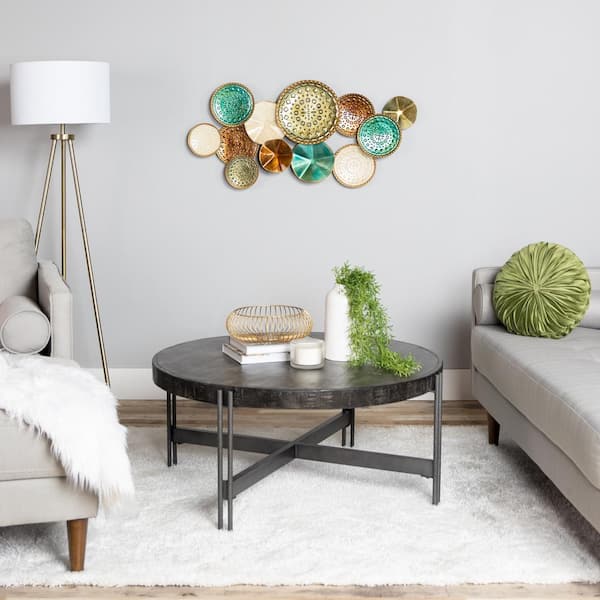The image shows a cozy, well-furnished room with a light gray wall complemented by wood trim and a wooden floor. A soft, fur-like white rug lies on the floor, adding a touch of warmth. The room features a charcoal gray coffee table adorned with a white planter overflowing with green leaves that spill gracefully onto the table. Also on the table, there is a white candle and an amber-colored candy jar resting on two reading books.

To the left of the coffee table is a plush gray chair paired with a matching gray ottoman. Draped over the chair is a fuzzy white blanket. A brass lamp with a white lampshade stands nearby, illuminating the space. On the right side, there's a grey cloth sofa, part of which is visible, adorned with a round olive green pillow featuring a floral pattern.

The walls are decorated with a collection of teal, yellow, and other colorful plates, creating a vibrant, linked pattern. The room also features a unique white lamp with gold legs, adding an elegant touch to the overall aesthetic.